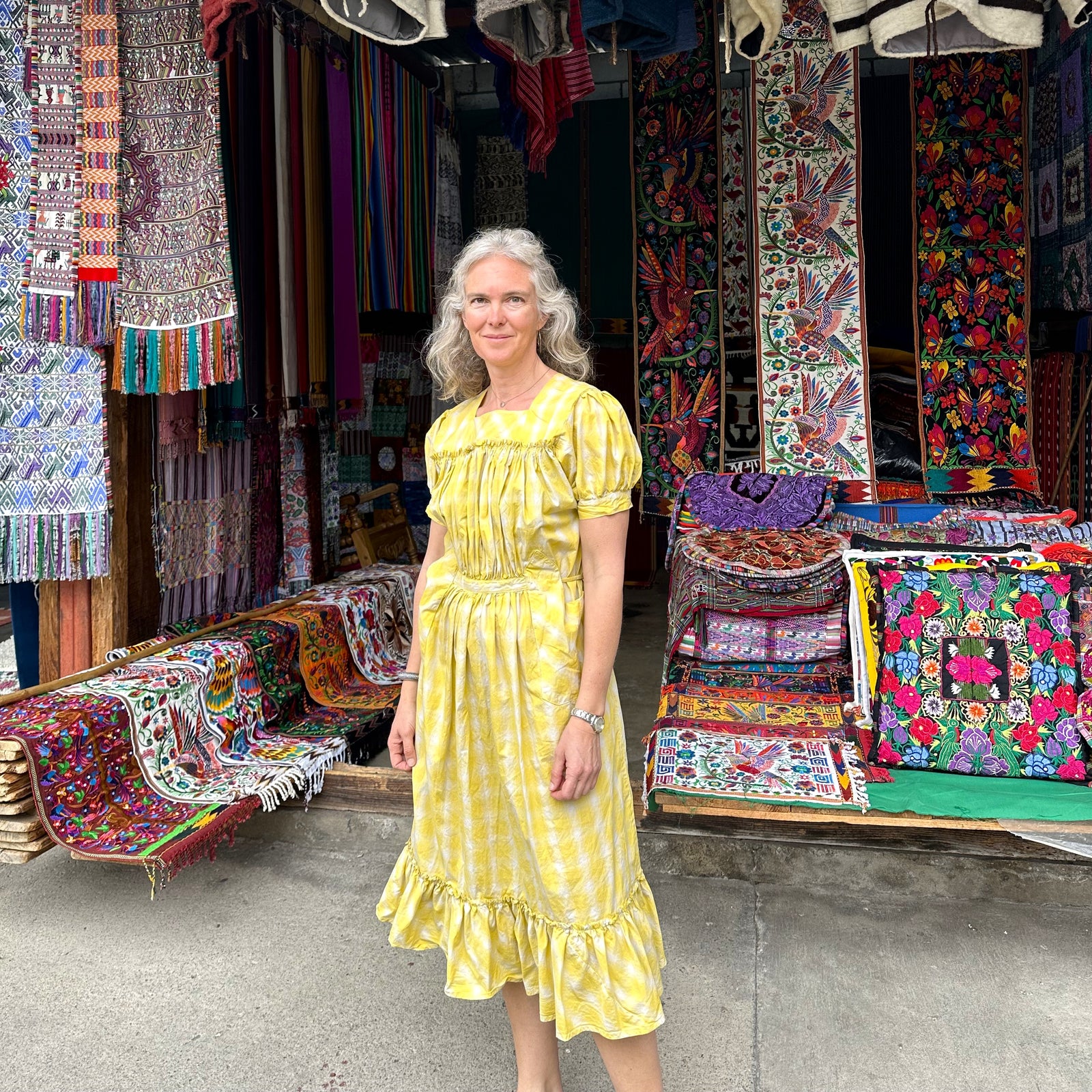In this outdoor scene, an attractive Caucasian woman with gray shoulder-length hair is posing amidst a vibrant display of woven rugs and blankets. She is modeling a short-sleeved, yellow and white checkered ruffled dress that gathers at the waist and has a frill at the bottom. The woman is accessorized with a wristwatch on her left hand and a bracelet on her right hand. She stands on a concrete surface, surrounded by colorful rugs that adorn tables and hang from ceilings and walls. The rugs are ornate, featuring flowers, birds, and intricate designs reminiscent of Indian blankets. To the left and right of her are benches covered with more of these vivid rugs, and in the background, the area appears to dim, resembling the deeper recesses of a fabric shop. Notably, one of the rugs hanging to the right features a repeating pattern of a hummingbird.